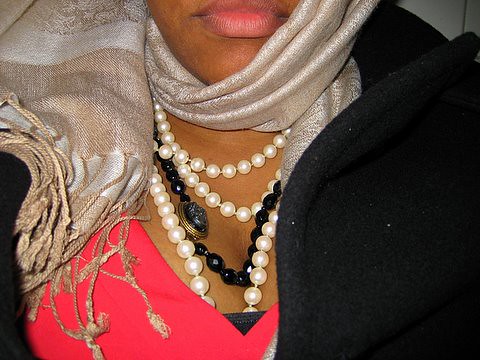This image features the lower part of a woman's face, from her lips down, with a prominent chin wrapped in a tan and off-white fringed scarf. The scarf is draped around her head and over her right shoulder. She is dressed in a pinkish-red blouse with a plunging neckline and a black jacket on her left shoulder. Around her neck, she wears multiple strings of beads, including white and black ones. The background appears to be a gray wall.